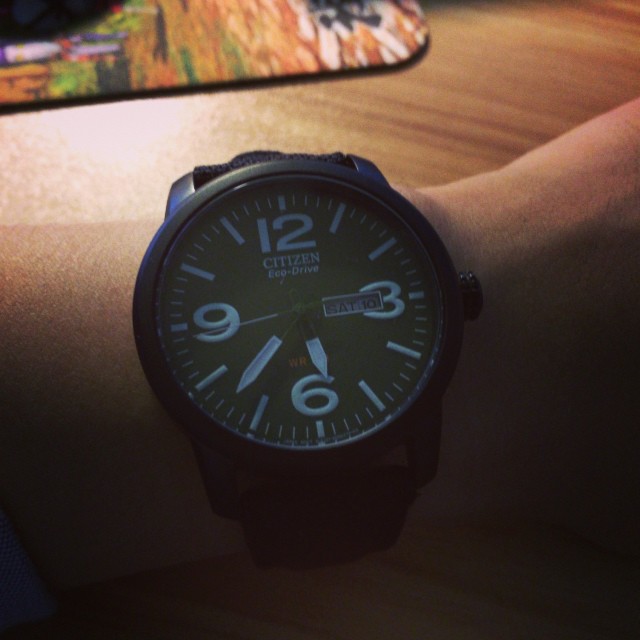In this close-up image, a man showcases his Citizen Eco-Drive watch, featuring a classic design with a rubber or fabric strap. The watch boasts an old-fashioned aesthetic, highlighted by its white, neon-like, possibly glow-in-the-dark numerals. Prominently displayed are the numbers 12, 3, and 6, while the time reads 5:37. The watch is likely held in the man's left hand, which is resting on a table surface, offering a clear and detailed view of the timepiece from a near angle.